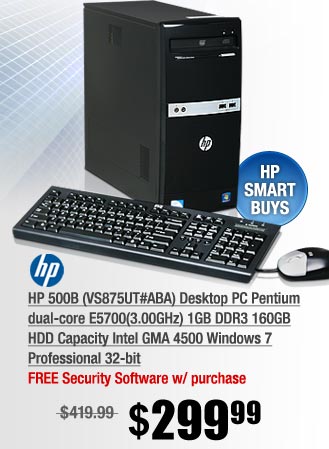**Detailed Caption:**

In this vintage digital advertisement, the upper left background features a light gray square pattern. The left and bottom parts of the image are predominantly white. The focal point is an older HP black desktop system. The front panel sports a gray stripe with a circular HP logo at its center. Accompanying the system is a black keyboard with white lettering and numbering, complemented by a mouse situated to the right; the mouse is equipped with gray push buttons and a scroll wheel.

Positioned above the keyboard, to the right of the desktop case, is a blue circle with the text "HP SmartPies" in white. Beneath this, on the left side of the ad, the blue HP logo prominently stands out, followed by the model name "HP 500B" in black text. The ad lists additional specifications: "HP Desktop Pentium 2 Core, E5-5700, 3GHz, 1GB DDR3, 160GB HSD Capacity, Intel GMA 4500, Windows 7 Professional 32-bit." Options for "Blue or Red" colors are also mentioned, along with a note about free security software included with the purchase.

The original price of $419.99 is crossed out in gray, replaced by a striking new price of $299.99 in bold black print. This discount highlights the perceived value of the system at the time, despite its now modest specifications like 1GB of RAM.